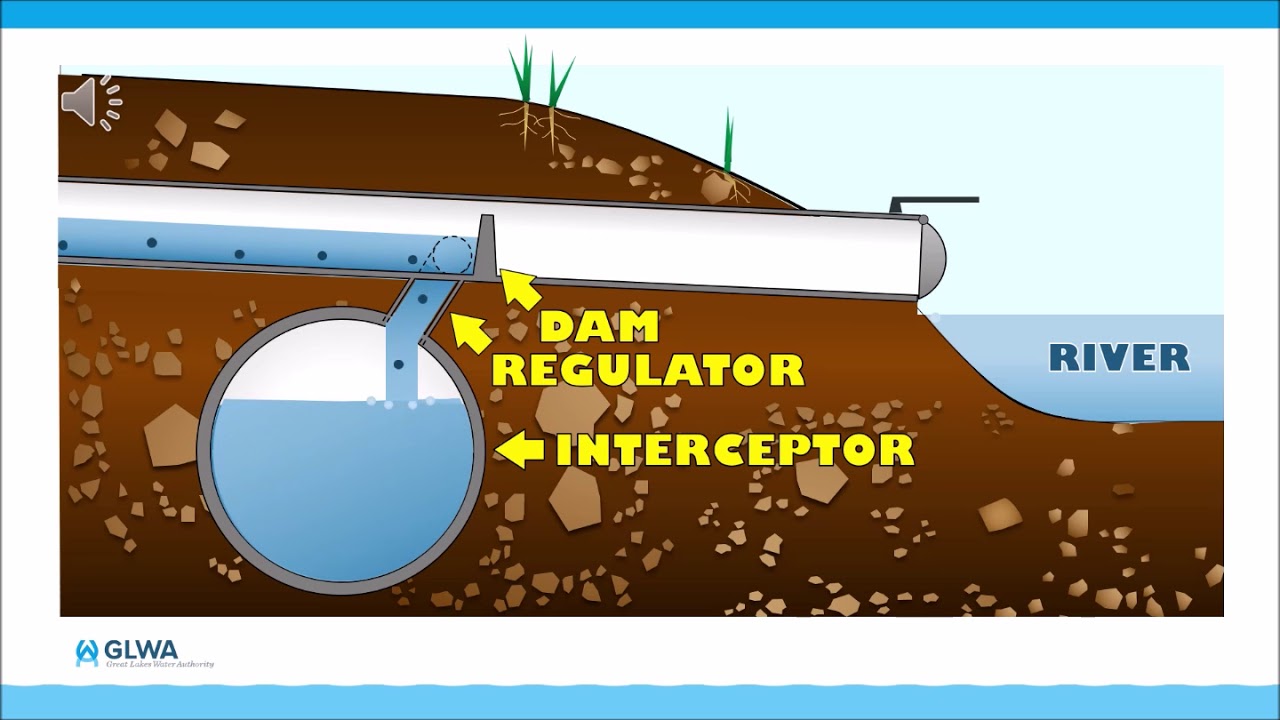The image depicts an informational diagram of a dam regulator system, positioned within a white background bordered by blue at the top and bottom edges. On the right side, a light blue area represents the sky, above a darker blue river, which is labeled "River." 

A white pipe extends across the image from the left towards the middle, intersecting with a blue section containing dark blue dots, marked "dam." Continuing rightward, the pipe transitions towards a vertical line labeled "Regulator," which descends into a circular section colored white on the upper half and blue on the lower half, labeled "Interceptor." 

The surrounding landscape is illustrated with a brown landmass, indicating soil, embedded with light yellow stones or rocks. Green foliage tops the embankment, which slopes downward on the right side and curves upwards on the left. 

Additional elements include yellow text and arrows pointing to various parts of the system, providing labels for the pipe, dam, regulator, and interceptor. A small blue icon in the bottom left corner bears the inscription "GLWA," and a speaker icon is positioned at the bottom right corner.